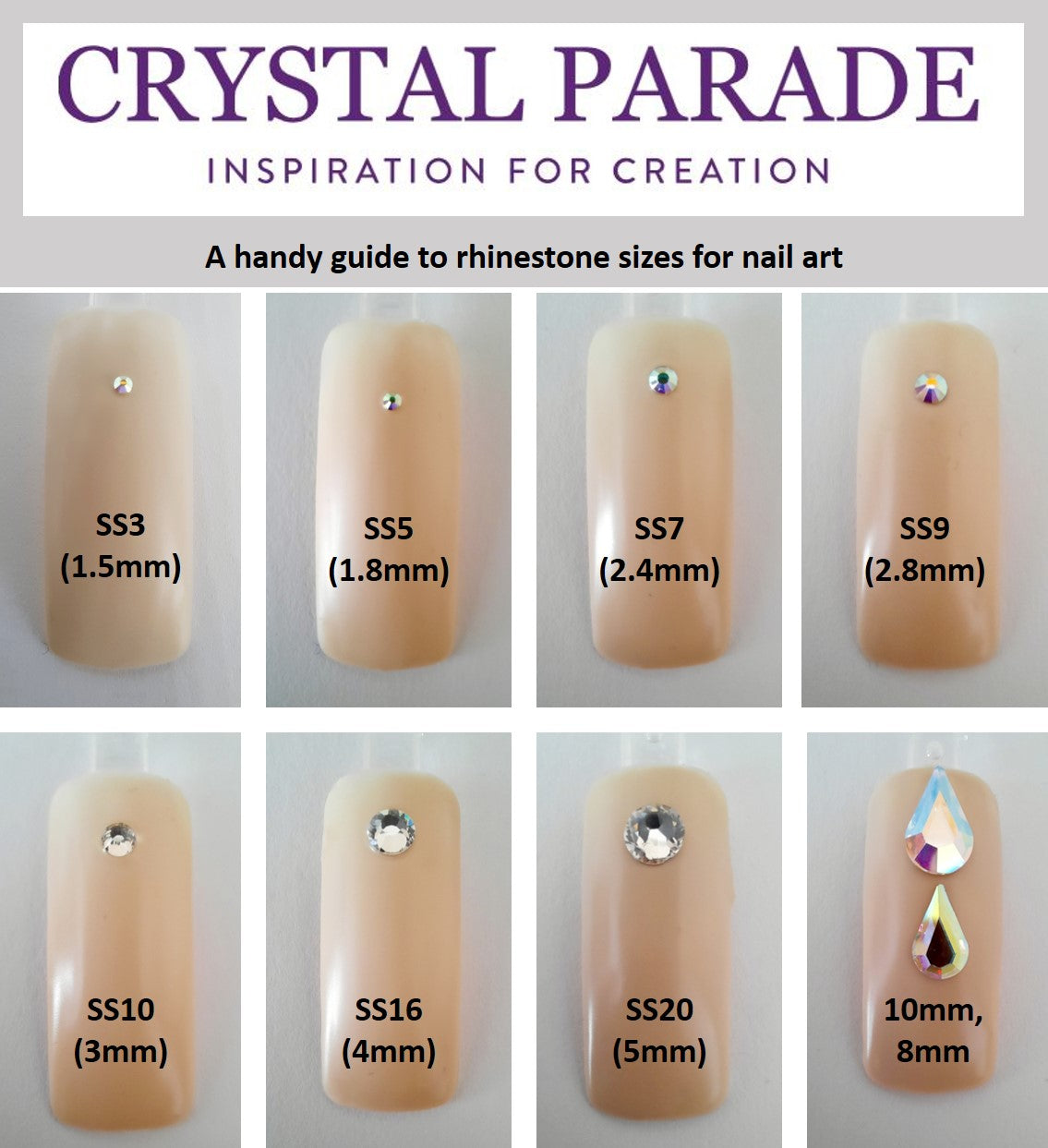This image serves as a detailed guide for selecting rhinestones for nail art, provided by the brand "Crystal Parade," known for their tagline "Inspiration for Creation." At the top, set within a white box, the text is written in purple, reading "Crystal Parade Inspiration for Creation." Beneath it, black text on a gray background states, "A handy guide to rhinestone sizes for nail art."

The guide features a grid layout with four columns and two rows, showcasing eight artificial nails painted a soft beige color. Each nail displays a rhinestone of different sizes to help visualize their dimensions. Starting from the upper left corner:

1. SS3, 1.5 millimeters
2. SS5, 1.8 millimeters
3. SS7, 2.4 millimeters
4. SS9, 2.8 millimeters

On the lower row:

5. SS10, 3 millimeters (noted previously as SS8)
6. SS16, 4 millimeters
7. SS20, 5 millimeters
8. Two teardrop-shaped crystals, one 10 millimeters and the other 8 millimeters, with a rainbow sheen.

This visual aid effectively demonstrates the relative sizes of different rhinestones, making it a useful reference for nail art enthusiasts.